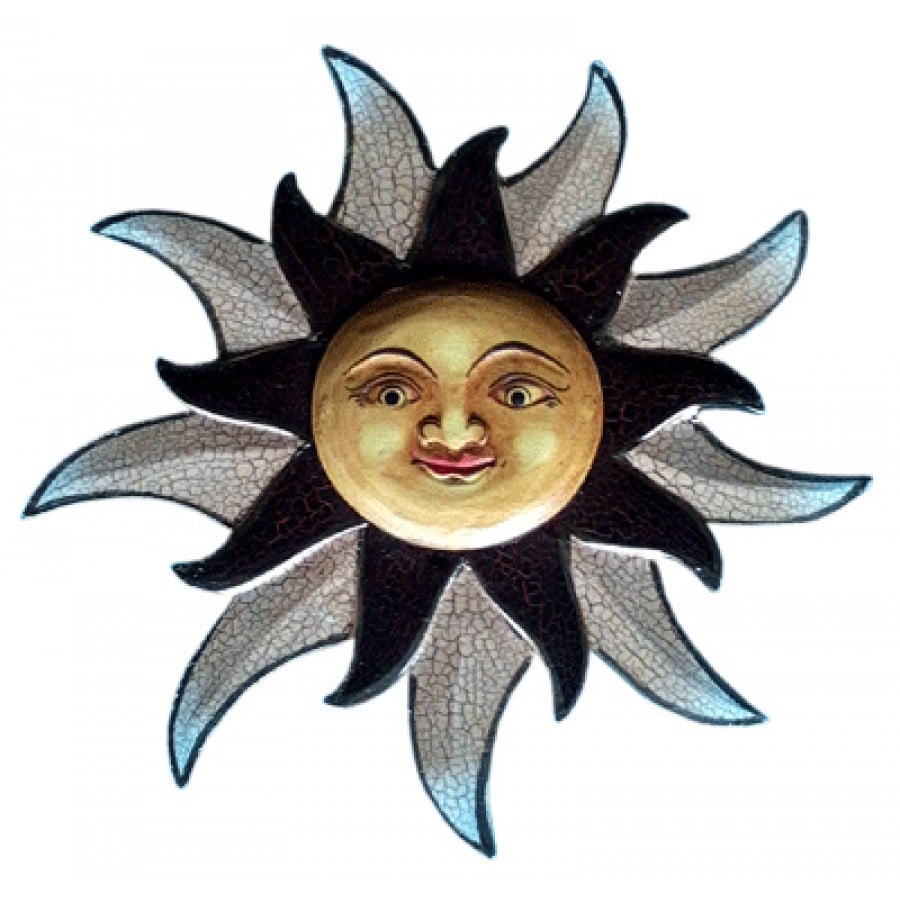This image is a detailed, stylized drawing of a fanciful sun with human-like features, reminiscent of illustrations from a children's book or comic. The central celestial body is a beige sun with a slightly irregular shape, sporting bluish eyes, red lips, a flat nose, and eyebrows. The sun's mouth is turned up into a smile. Surrounding the sun’s face is a series of decorative rays: the first layer consists of about eight dark black fins, each outlined in black, resembling sun rays. Behind these black fins are a larger group of approximately eight bluish or grayish-white fins, also outlined in black. These fins are slightly offset, creating a layered effect that makes the rays look superimposed. The entire composition is rich in color and detail, but it lacks any background, focusing solely on the whimsical and intricate representation of the anthropomorphic sun.